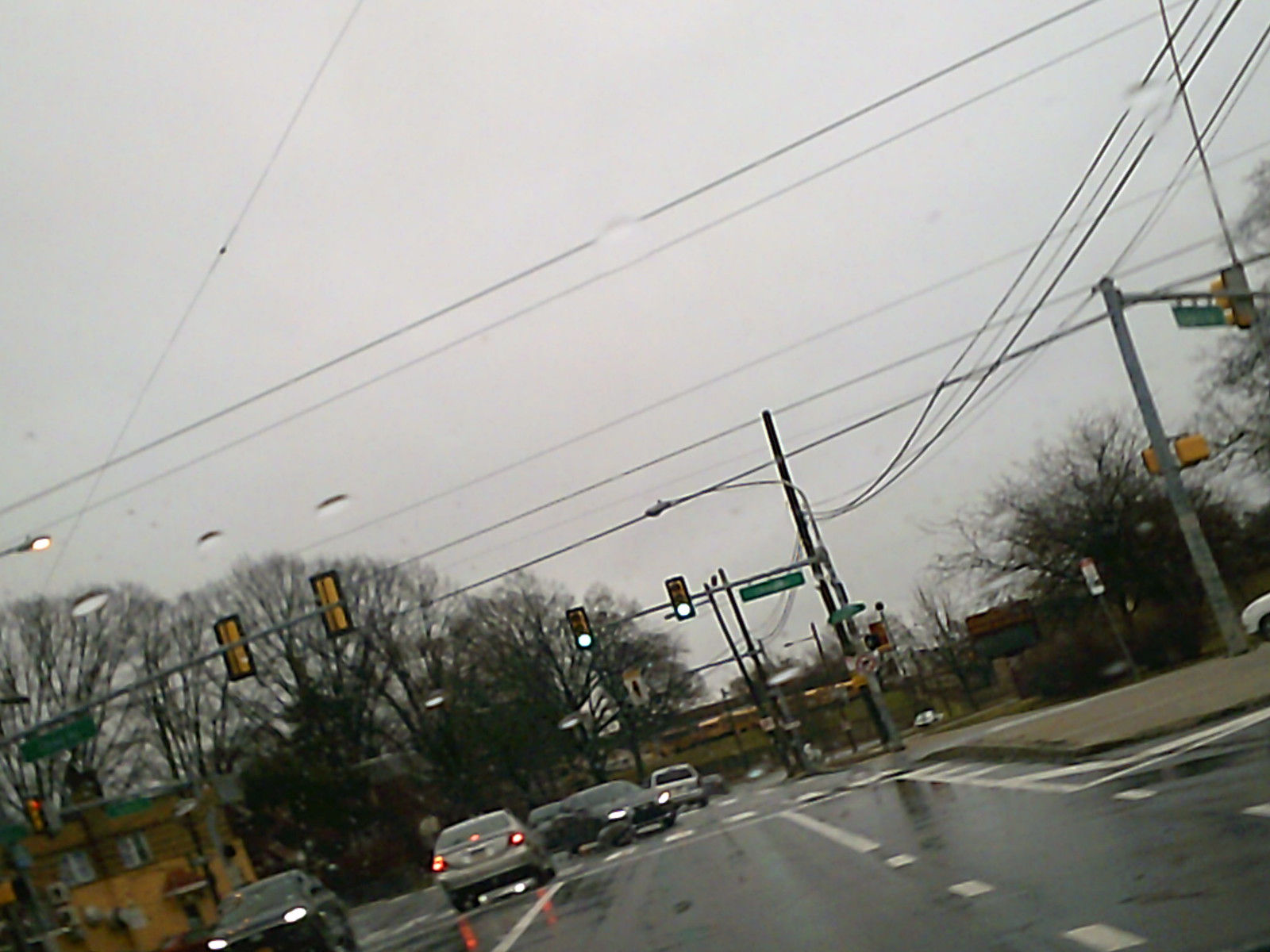A photograph captures a rainy street scene from an inside-the-vehicle perspective, giving the image a noticeable tilt with the street slanting lower on the left and higher on the right. The wet pavement gleams under the overcast sky, suggesting recent or ongoing rain. The visible section of the road appears to have two lanes flanked by a shoulder and a central concrete island. Above these lanes, a traffic light shines with white illumination, inferred to be green due to the low-contrast lighting. A green street sign hangs nearby, though its text is indiscernible.

Reflecting a wintry atmosphere, the barren branches of deciduous trees stretch across the background. Most vehicles in the scene are a dull gray, with the exception of one displaying vivid red taillights and two others with glowing headlights. On the left side of the image, a gold-hued building stands out, while a cluster of yellow school buses can be faintly seen in the distance, positioned in a line. The overall ambience of the photograph conveys the cold, wet, and somewhat dreary impression of a winter day in an urban environment.